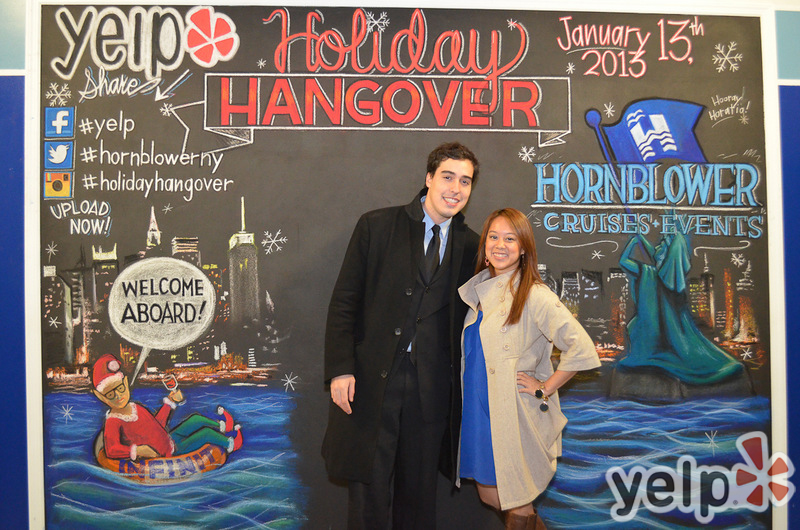In the image, a smiling couple stands centered in front of a black chalkboard sign with a white border. The man, positioned on the left, is tall with brown hair and dressed in a black suit, blue collared shirt, black tie, and a long black trench coat. The woman to his right, with long brown hair, wears a blue dress and a tan trench coat, smiling with her hand on her hip. Above them, in red, fancy lettering, the sign reads "Holiday Hangover," while "January 13, 2013" is written to the right in black lettering. On the left side of the sign, the word "Yelp" appears in black bubble letters accompanied by a flower symbol. Below this, various social media hashtags (#Yelp, #HornblowerNY, and #HolidayHangover) and logos are displayed, encouraging viewers to upload photos. Additionally, a small cartoonish figure at the bottom left with a white speech bubble says "Welcome Aboard." The festive theme and celebratory elements suggest a promotional event by Hornblower Cruises and Events.